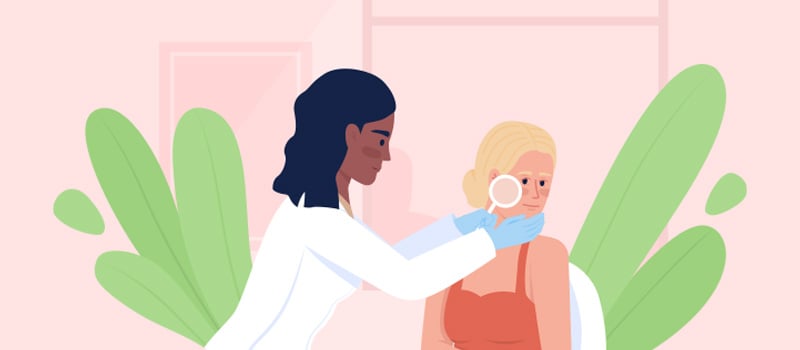In this computer-animated, illustration-like image, a female doctor with shoulder-length black wavy hair, dark complexion, and blue gloves is standing on the left side. She is dressed in a white coat and holding a magnifying glass-like object, attentively examining the face of a female patient. The patient, with her blonde hair pulled back, blonde eyebrows, and dark eyes, is seated in a white chair wearing a red tank top. The setting is brightly highlighted by a vivid pink background, and lush green plants with large leaves are positioned on either side, adding to the visual appeal of the scene. The overall composition, reminiscent of a cartoon or comic strip, is notably wider than it is tall, and the doctor's meticulous focus on the patient's face creates a scene of attentive medical care and examination.